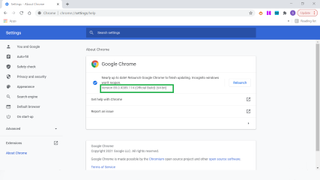The image depicts a small and slightly blurry screenshot of the Google Chrome browser's settings page. Despite the blurriness and small size, the Google Chrome interface is discernible. The top of the screen clearly states "Google Chrome," and directly below this heading, a particular setting is highlighted with a green rectangular box, drawing attention to it. The left-hand side of the screen showcases a vertical menu of settings against a light grey background. The top right corner of the screen features several small icons of varying colors: yellow, purple, blue, grey, and another shade of purple, followed by a button outlined in red with red text inside. A prominent blue banner runs across the top portion of the screen, indicating that the user is in the settings section and can delve deeper into various options. The main focal point of the image is the green-highlighted setting, signifying its importance.